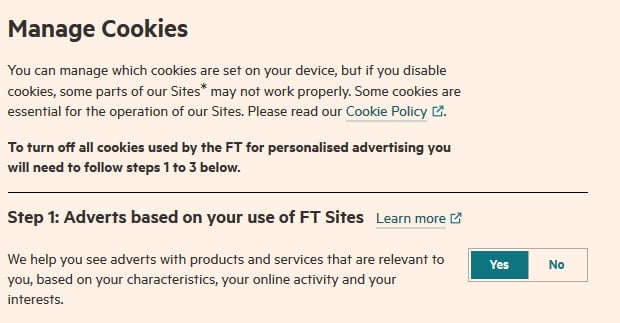This screenshot mainly features a large, peach-colored rectangle with the header "Manage Cookies" prominently displayed at the top. Below the header, there's a paragraph explaining that users can control which cookies are set on their device. It cautions that disabling certain cookies might affect the proper functioning of parts of the website, emphasizing that some cookies are essential for the site's operation. The paragraph ends by advising users to read the full cookie policy.

Following this, a bold statement informs users that to turn off all cookies used by the Financial Times (FT) for personalized advertising, they need to complete the steps listed below. A black horizontal line visually separates this section from the subsequent content.

Under the black line, there's the heading "Step 1" with the subheading "Adverts based on your use of FT sites." A clickable button labeled "Learn More" appears next to this heading. Below, a sentence explains that FT uses cookies to show users advertisements relevant to their characteristics, online activity, and interests. Adjacent to this explanation, there is a toggle button allowing users to opt in or out by selecting "Yes" or "No." Additionally, the screenshot includes built-in links to the detailed cookie policy as well as a separate page for learning more about these advertising practices.